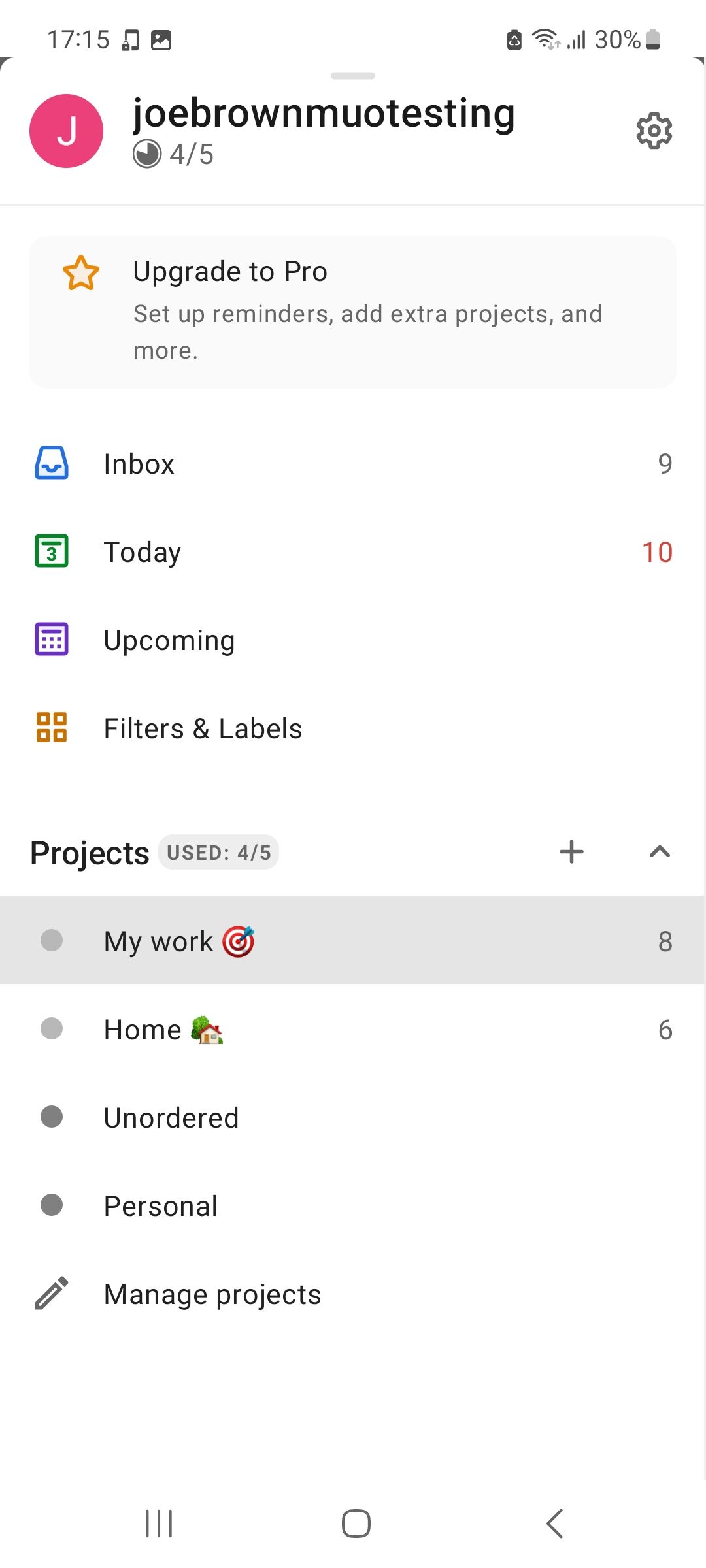### Descriptive Caption for the Image:

The vertical image appears to be a screenshot taken from a smartphone. The background predominantly features a white shade, seemingly derived from a computer screen. A thin gray line runs down the right-hand side, serving as the screen's border, with no borders present on the other sides.

In the upper-left corner, the time is displayed in military format as "17:15." Adjacent to this, there are two icons: a photo icon and a padlock icon. Shifting to the upper-right corner, several other icons are visible, including the WiFi indicator, signal strength bars, and a battery icon showing 30% charge. 

Below this top section, a reddish circle featuring a white "J" within it reads "Joe Brown Muau testing." To the right of this area, it displays "4 out of 5," along with a settings icon. Nearby, there is a small box containing a star icon, with a message promoting an upgrade to a pro version that includes additional features like setting up reminders and adding extra projects.

Further down, the screen shows an organization layout with categories such as "Inbox" showing nine items, "Today" with ten items, and a section labeled "Upcoming." Each of these categories is accompanied by its respective icon. Additionally, it mentions "Projects used: 4 out of 5" with a plus sign beside it. Beneath this, listed projects include "My work" identified by a bullseye icon with eight items, and "Home" labeled with a home icon containing six items. 

Lastly, there are sections named "Unordered," "Personal," and "Manage Projects," each sporting either a circular icon or a unique symbol.

At the bottom of the screen, various other icons are visible, though they are not explicitly described in detail.

This comprehensive representation captures the essence and contents of the screenshot.